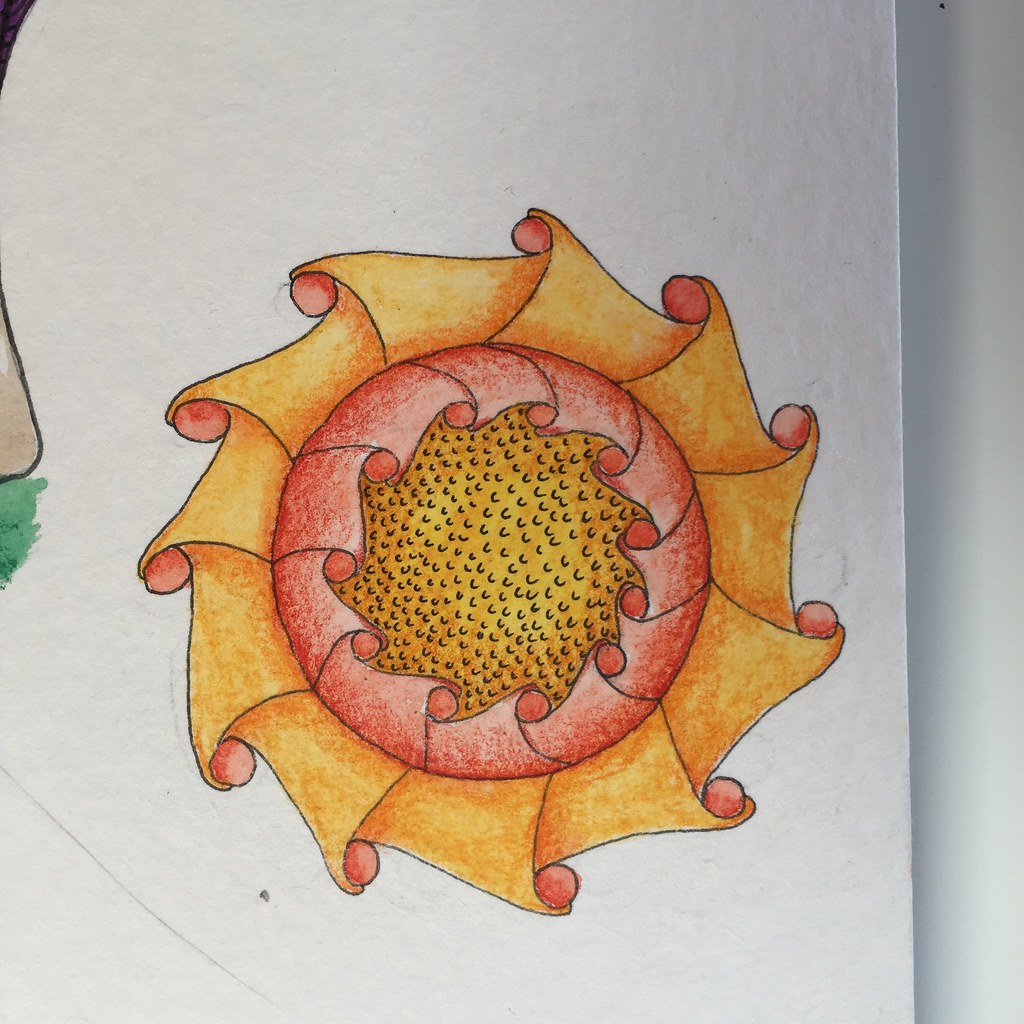The photograph captures a hand-drawn image on a piece of textured white paper, which is held slightly above a smooth white surface in the background, casting a soft shadow. The artwork itself appears to be crafted using a black ballpoint pen for the intricate linework, with additional shading rendered in crayon. The background of the drawing seems to be filled in with colored markers. The design is circular, featuring multiple petal or scroll-like curves extending outward. At the center of the circle, a dotted texture suggests a raised or bumpy surface. Surrounding this central area, there is a row of red curved petal-like shapes that curl inward. Beyond this, a layer of orange, similarly curled and raised textures, fans outward from the core, creating a vibrant and dynamic composition.